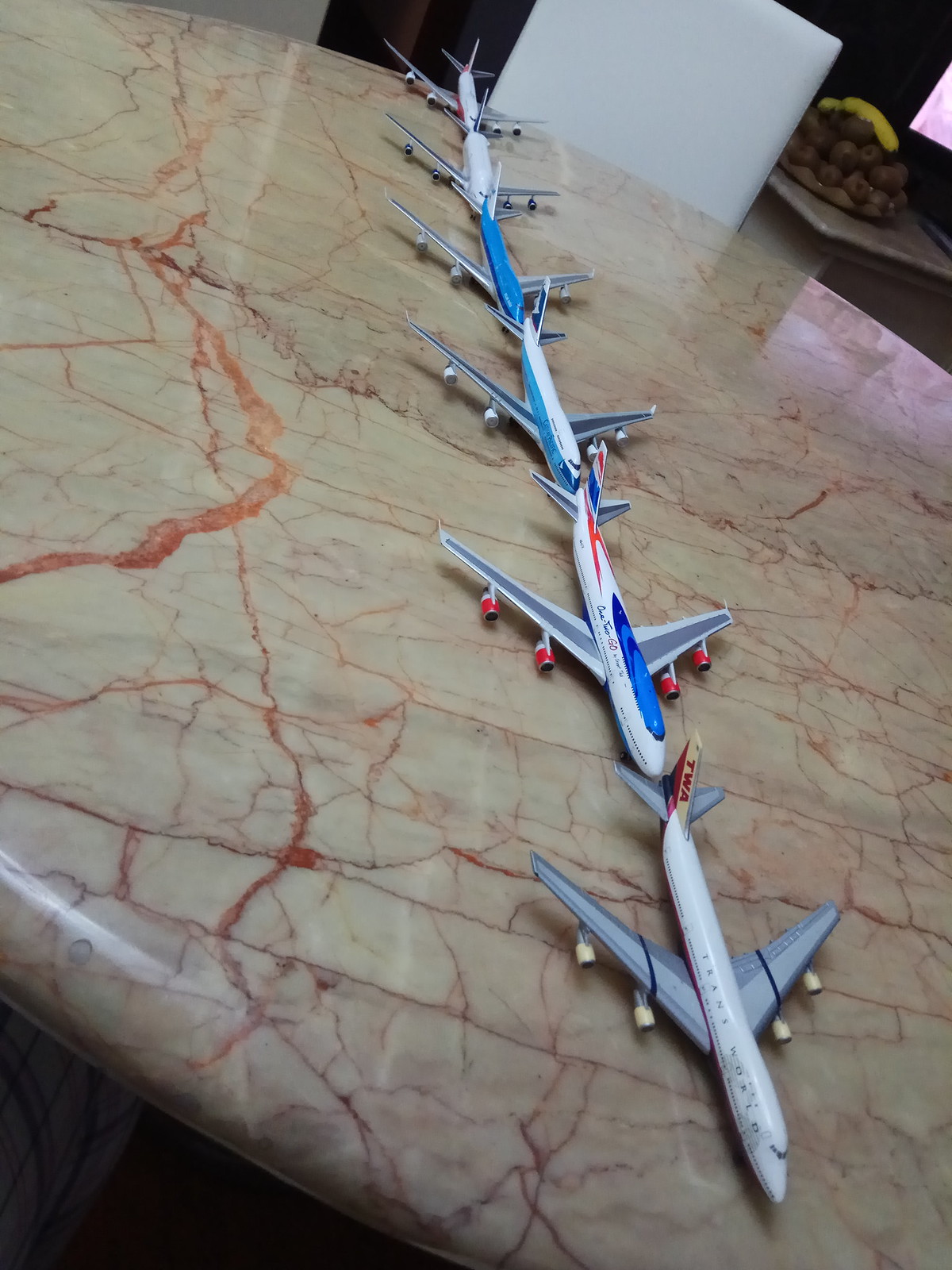The image captures a realistic and detailed scene set indoors, featuring a circular marble table with intricate patterns of crimson, orange, and purple swirls on a tan background. This table, about 8 to 10 feet in diameter, serves as the focal point of the photograph. Arranged neatly in a vertical line down the center of the table are six model jetliners of various colors. The first plane at the bottom of the image has a white fuselage and gray wings, branded with "TWA" on its tail. Moving upwards, the following planes include a white body with a bright blue top and gray wings, a blue body with blue wings, a plane with alternating white and blue colors, and two completely white planes. In the background, to the upper right, a white box and a bowl of brown fruits, possibly kiwis, with two bananas on top, can be seen. The overall composition of the image is slightly tilted, adding a dynamic element to the carefully arranged scene.